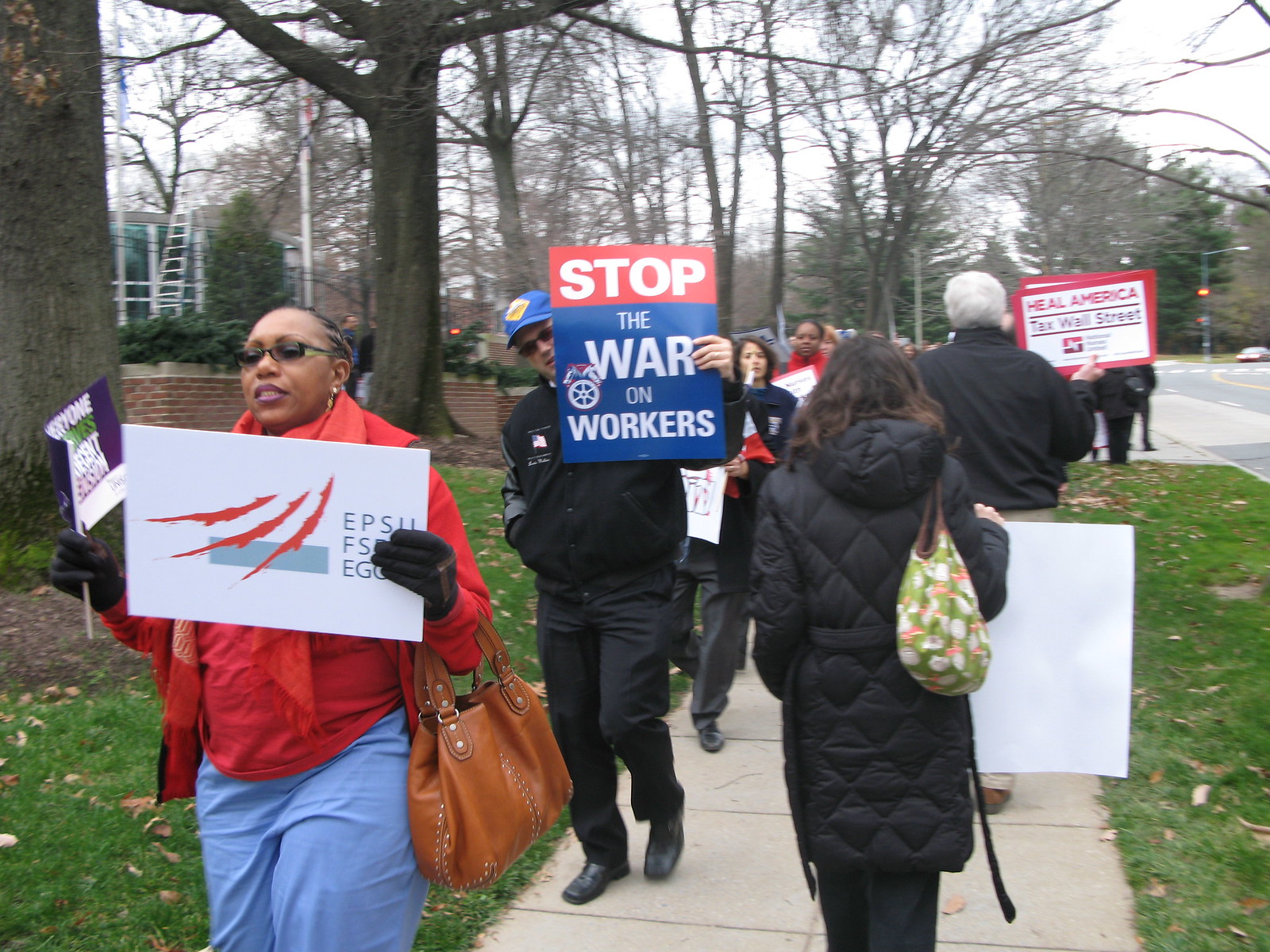The photograph captures a small protest taking place on a sidewalk in what appears to be a residential neighborhood. A diverse group of demonstrators, including both white and black individuals, hold various signs and march in single file toward the camera while some participants walk away, their signs unseen. Prominent signs include one with red at the top reading "Stop the War on Workers" in white and blue, and another that reads "Heal America, Tax Wall Street." The main street alongside the protest remains completely open to traffic, with a car visible in the background. The scene, set in the middle of the day, feels cold, suggested by the bare trees devoid of any leaves and people dressed warmly. Hints of nearby houses further emphasize the residential setting.